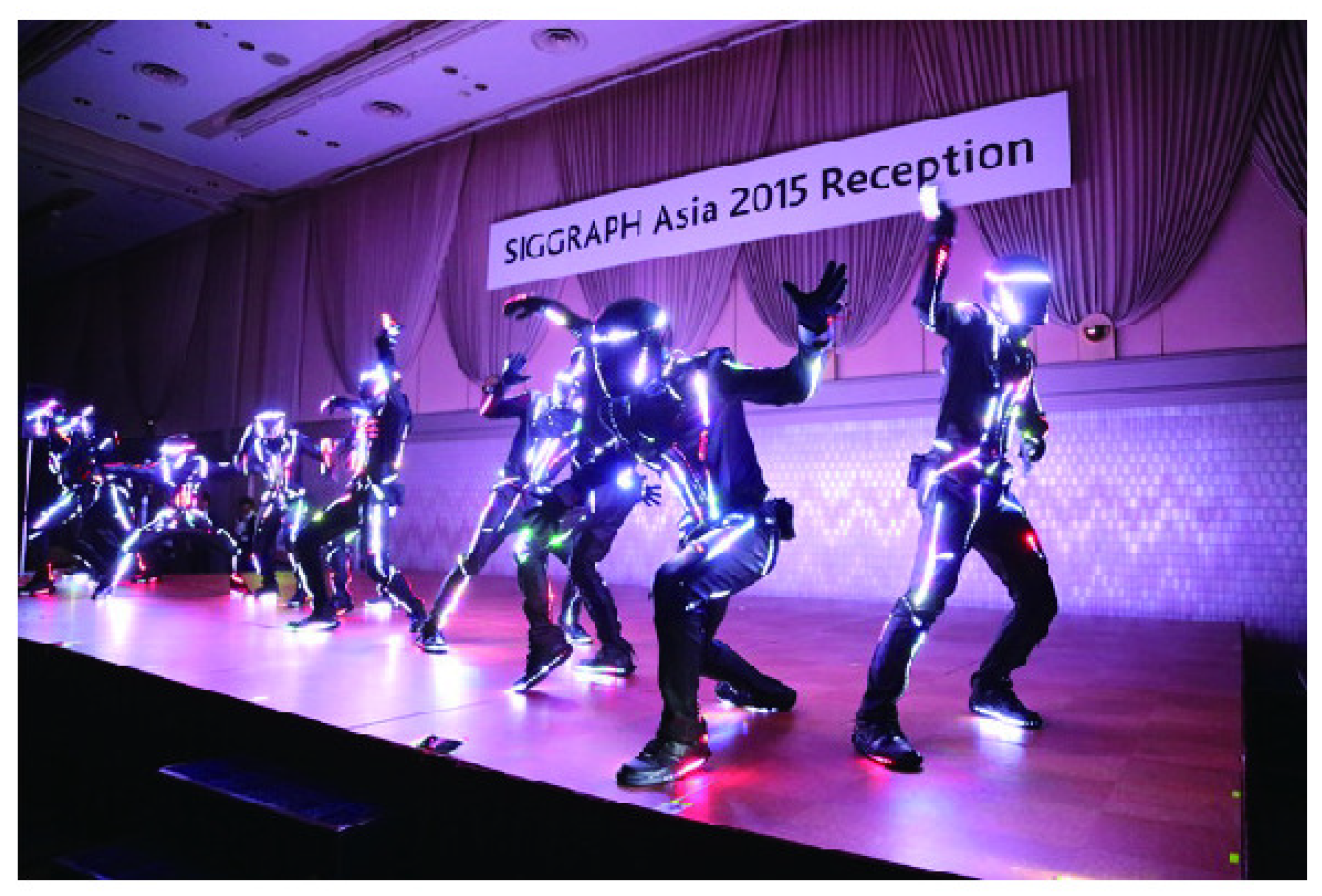The image features nine dancers on a wooden stage, all dressed in full black suits that cover their bodies, faces, and hands. Their outfits, which resemble motorcycle suits, are adorned with lights, with illuminated lines visible on their thighs, chests, arms, and shoes, as well as their helmets. The stage is illuminated with purple and red lighting, creating a vibrant effect. Behind the dancers is a large sign that reads "SIGGRAPH ASIA 2015 RECEPTION" in black lettering on a white background. The backdrop features lined, textured curtains that appear purple in the lighting, with a brick wall partially visible at the bottom. The dancers are either striking various poses or mid-dance, adding dynamic energy to the scene.